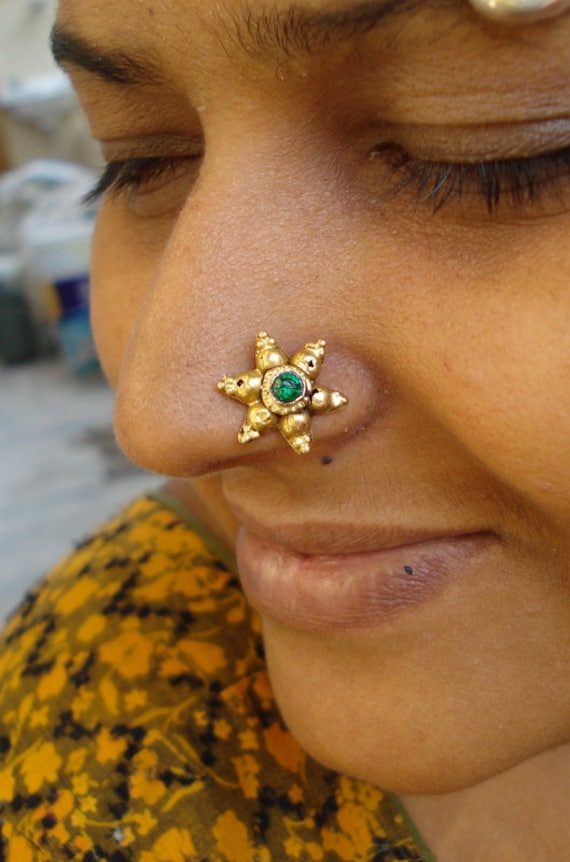This close-up photograph features a woman's face, approximately 35 years old, who is turned slightly to her right and looking downward. Prominently displayed on her left nostril is a large, gold star-shaped nose ring, adorned with a green gemstone in the center. The ring consists of six star points and occupies the entire nostril. Her dark brown eyelashes and light brown skin are visible, as well as a hint of an eyebrow barbell in the top right corner of the image. The background is blurred, revealing just a hint of a building structure and muted tones of gray and white. The woman is dressed in a floral patterned top featuring muted colors like orange, black, green, and yellow. This close-up, highly focused image showcases the piercing jewelry in great detail while casting the background into an indistinct blur.